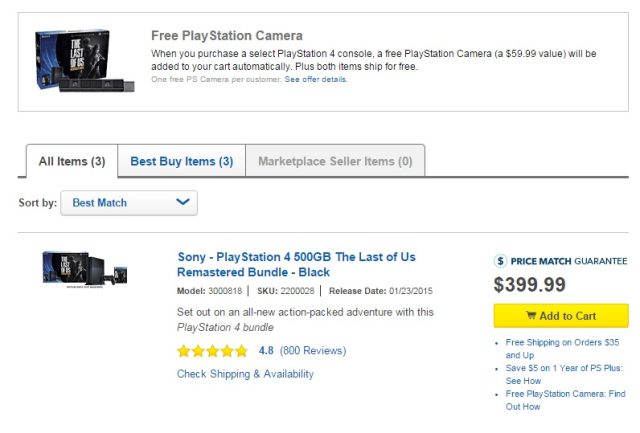At the very top of the page, a prominent outlined rectangle stretches across the entire width, serving as a banner. Inside this rectangle, on the left, is a picture of a PlayStation camera, next to a box featuring the cover image of the video game "The Last of Us." 

The title within the rectangle reads "Free PlayStation Camera," emphasizing the promotional offer. The text beneath the title explains: "When you purchase a select PlayStation 4 console, a free PlayStation camera (a $59.99 value) will be added to your cart automatically. Plus, both items ship for free." In a smaller, lighter font below, it mentions, "One free PS camera per customer. See offer details." The phrase "See offer details" appears in blue, indicating a clickable link.

Below this banner, a section for shopping options is introduced, featuring three tabs at the top. The first tab is labeled "All Items" with a "(3)" in parentheses, the second tab says "Best Buy Items" also with a "(3)" in parentheses, both written in blue, while the third tab, "Marketplace Seller Items (0)," is grayed out. The "All Items" tab appears to be selected. 

Beneath these tabs, on the left side, there's a "Sort By" option with a dropdown box showing "Best Match" selected in blue. A dividing line separates this from the content below.

The content showcases a product: a PlayStation 4 console. On the left, there's an image of a PlayStation 4 with "The Last of Us" game. In blue text, it reads: "Sony PlayStation 4, 500GB, The Last of Us Remastered Bundle in Black." Additional details include the model number, SKU number, and release date. 

A brief description follows: "Set out on an all-new action-packed adventure with this PlayStation 4 bundle." Then, a rating display shows five yellow stars with "4.8" written next to it, followed by "(800 reviews)." Below this, an option to "Check Shipping and Availability" is provided.

On the right side of the page, the header features a dollar sign inside a circle next to "Price Match Guarantee." The price is prominently displayed in black text: "$399.99." Directly beneath the price, a large yellow button with a shopping cart icon to its left reads "Add to Cart." Below this button, three clickable options are listed: "Free Shipping on Orders $35 and up," "Save $5 on one year of PS Plus: see how," and "Free PlayStation Camera: find out how."